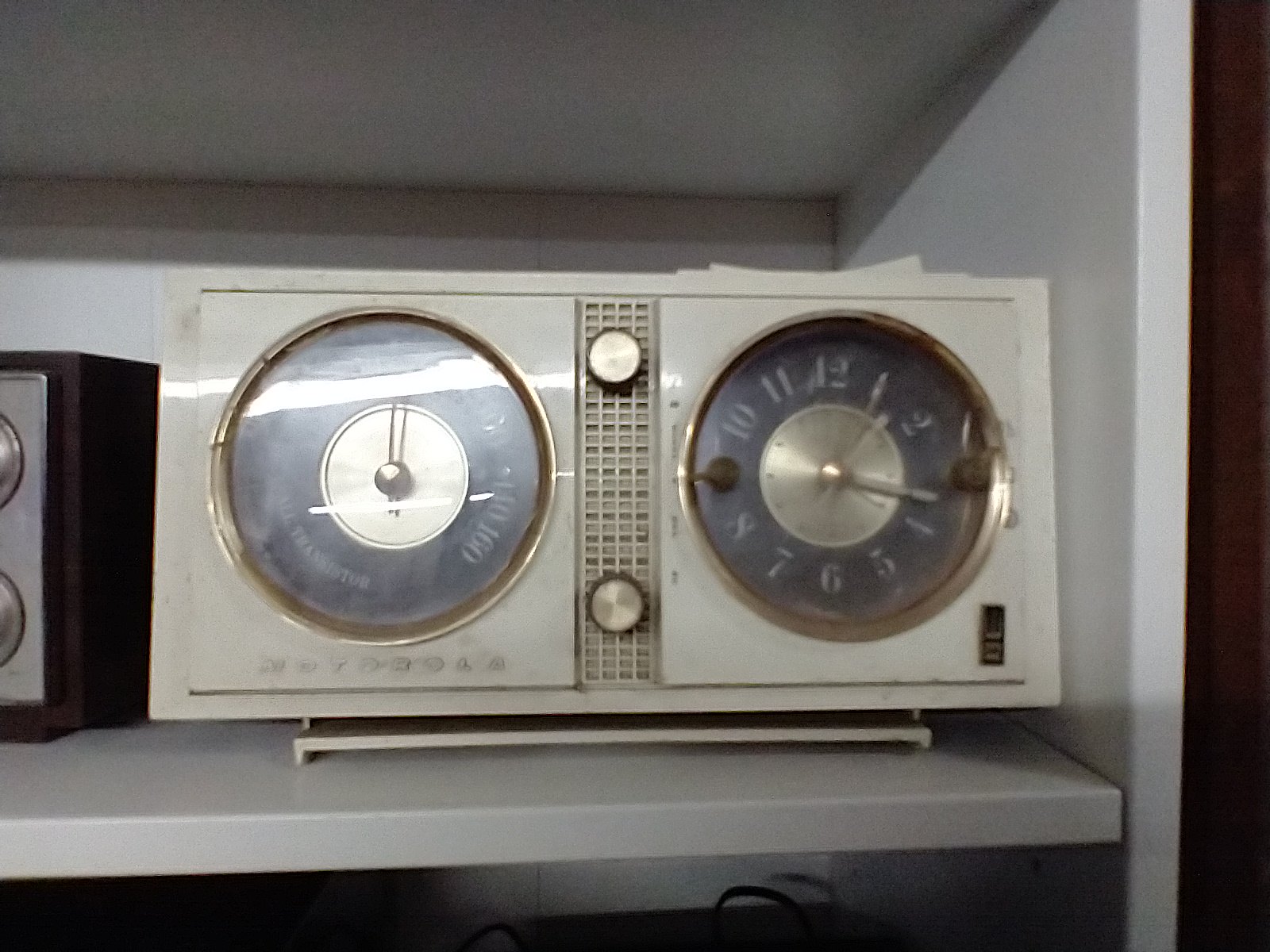This image features a mid-century modern style clock, positioned on a pristine white shelf. The clock's body is an elegant cream color and it boasts two circular faces. The face on the right-hand side indicates the current time, showing 1:17. The identity of the left-hand face is obscured by glare from the surrounding lighting, but it is likely a secondary function such as a thermometer. Central to the clock's design are two prominent knobs, one at the top and one at the bottom, which are flanked by intricate small rectangular details. This blend of functionality and sophisticated design from the mid-century era creates a nostalgic yet timeless piece.